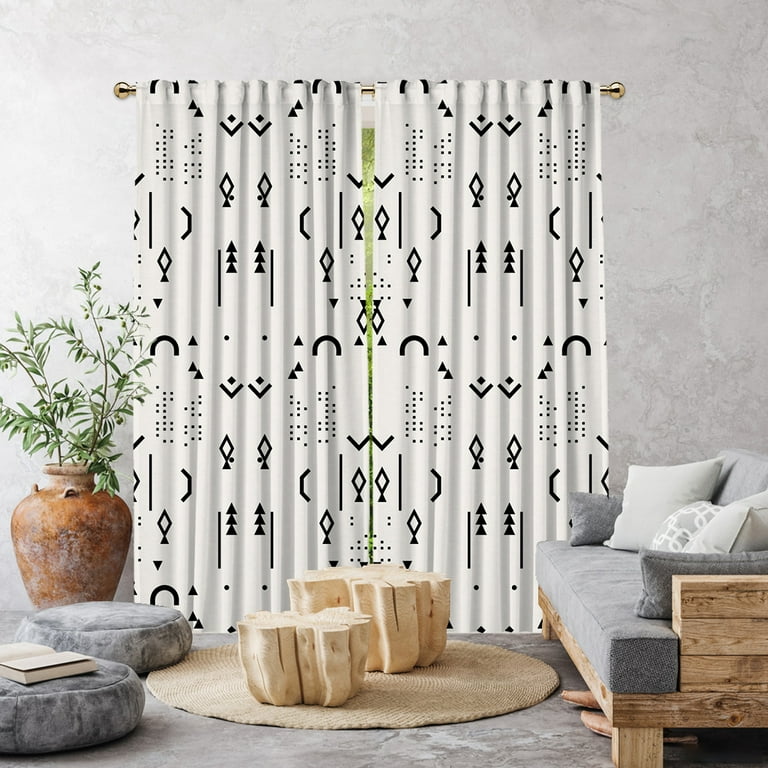This image depicts a rustic and inviting living area with various intricate details. The walls are a sophisticated grayish white, resembling a marble texture. Central to the room is a golden curtain rod adorned with white curtains showcasing a geometric pattern in black, and behind them, a touch of greenery peeks through. The centerpiece sofa is crafted from light-colored wood, featuring thick gray cushions complemented by a variety of gray pillows, some with delicate white lines. Resting on a brown rug are two wooden tables, fashioned to resemble logs with flat tops. The gray carpet hosts a straw-like beige round rug, adding a touch of warmth. Two gray round poofs, one holding a book, provide additional seating. To the left, a large ceramic planter with lush green leaves enhances the natural, cozy atmosphere. All these elements together create a harmonious and aesthetically pleasing living space.